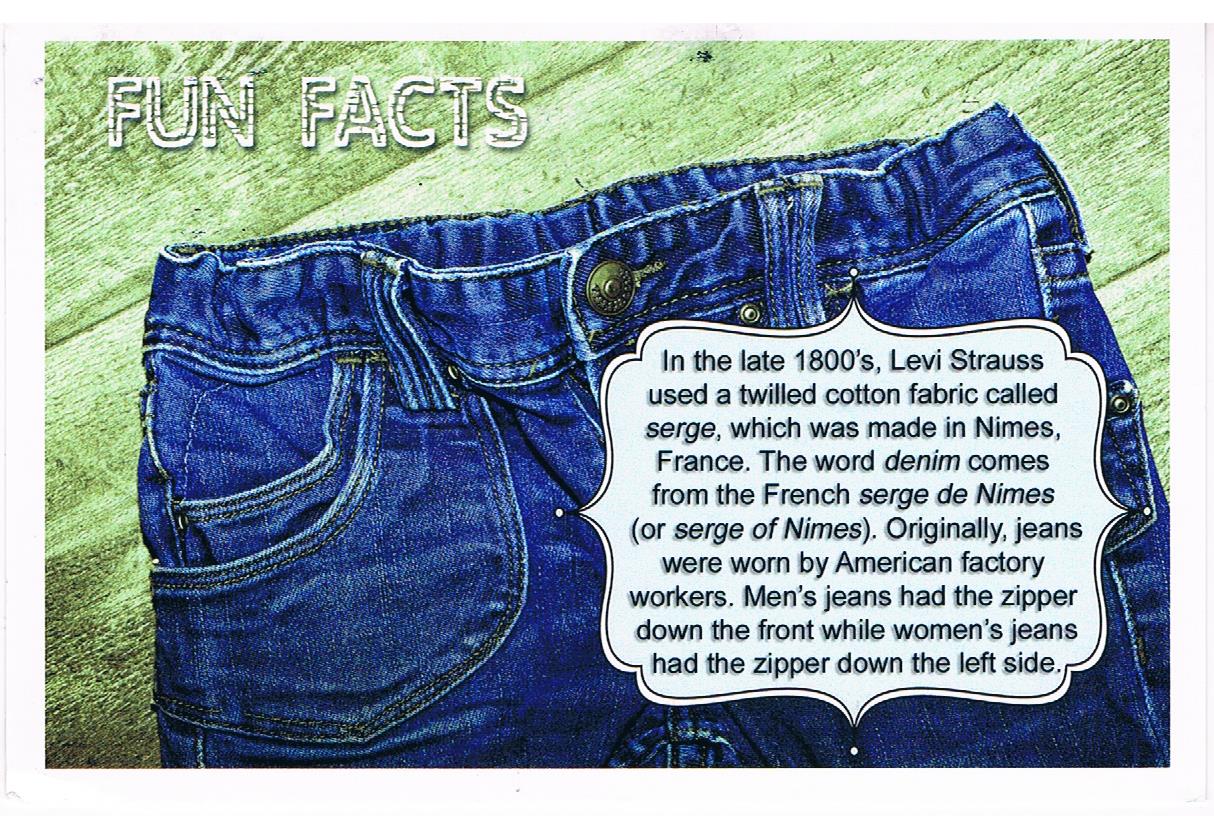This detailed photograph showcases a pair of blue denim jeans, displayed from the crotch up and buttoned at the waist, laying on a background of light green, diagonally arranged wood planks. The jeans sport visible belt loops and two pockets on the left side. Positioned in the upper left corner, the text "fun facts" is written in green with a white outline. Over the right side of the jeans, a white-bordered label with black text reads: "In the late 1800s, Levi Strauss used a twilled cotton fabric called 'serge,' which was made in Nimes, France. The word 'denim' comes from the French 'Serge de Nimes' or 'Serge of Nimes.' Originally, jeans were worn by American factory workers. Men's jeans had the zipper down the front, while women's jeans had the zipper down the left side." The overall image has a thin white border and is presented in a landscape orientation. The blue of the denim contrasts with the weathered white-gray hue of the wood background, giving the image a visually striking appearance as if saturation has been increased.